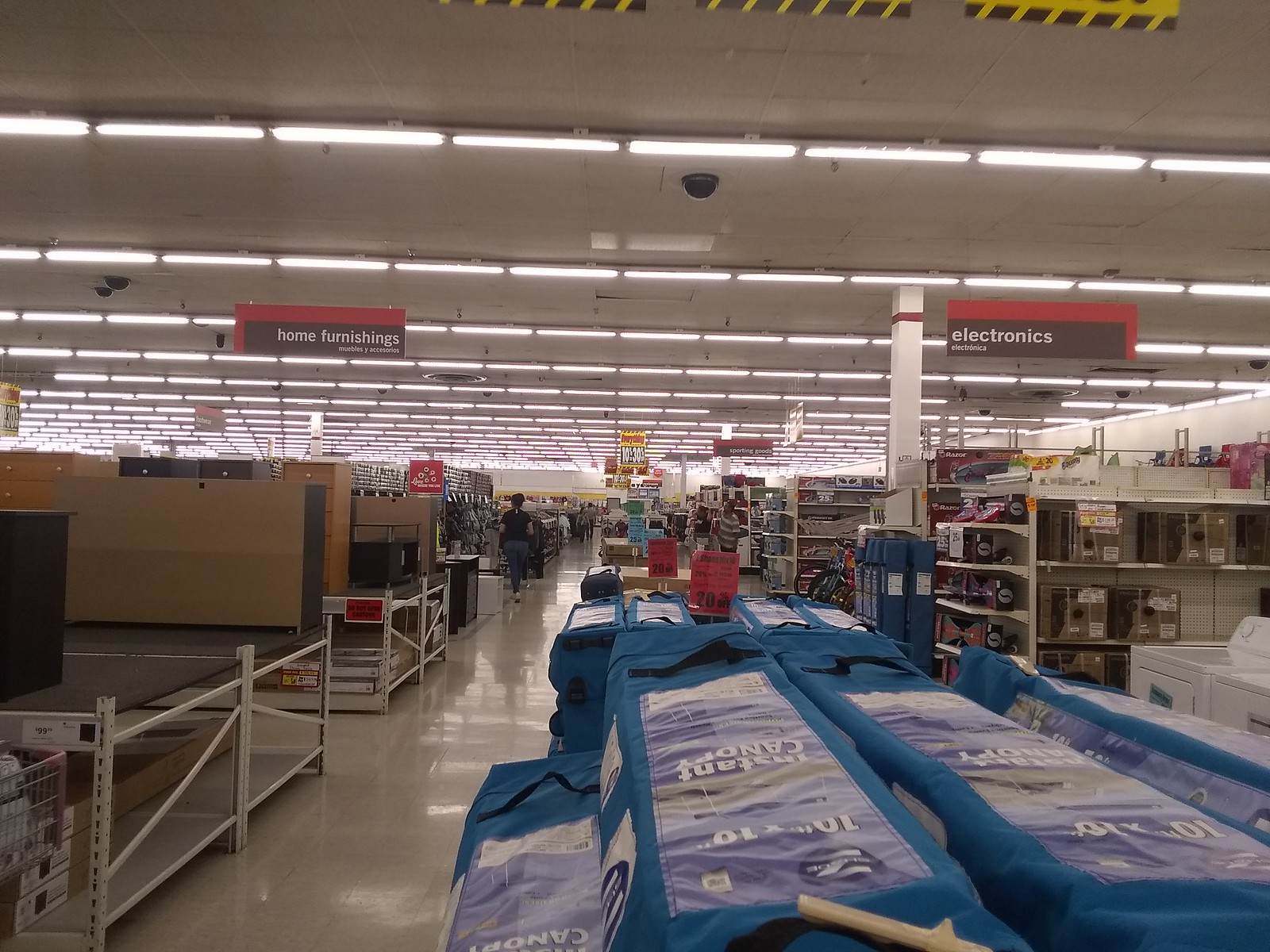This detailed color photograph captures the interior of a large superstore, potentially a Target, from the vantage point of a central aisle. Dominating the foreground is a stack of long, blue rectangular items, likely canopies or duffel bags, neatly arranged and displaying light blue coverings. On the left side, a mixture of light round furniture pieces stands atop elevated, white-colored scaffolding with a black top. Additionally, large furniture items in shades of black, dark brown, and chocolate brown are visible.

Adjacent to this furniture display is a section with light gray, reflective tile flooring, illuminated by horizontally aligned, rectangular fluorescent lights affixed to the light gray ceiling. Suspended from the ceiling are a few black security cameras. Shelves filled with various items extend into the background on both sides of the aisle, with the ones on the left appearing empty in the foreground but more populated toward the center.

Prominently, there are red signs hanging from the ceiling, one on the left indicating "home furnishings" and one on the right labeled "electronics" with small black rectangles. On the right side of the image, a white machine washer is visible among the shelves. A person dressed in a black shirt and black pants can be seen walking in the middle distance, pushing a cart beneath the "home furnishings" sign. This setup reflects the organized and vast layout typical of a department store, emphasizing the variety of merchandise available.